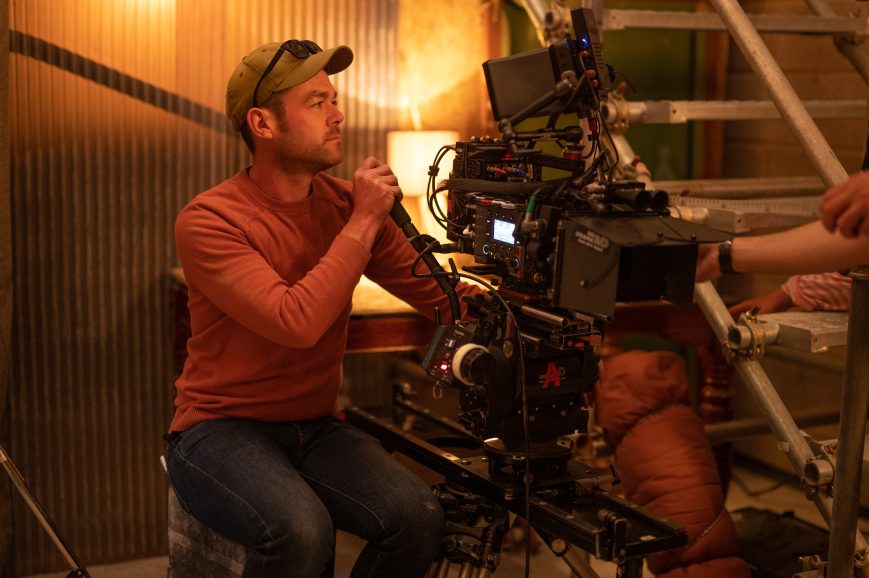In this image taken inside a studio, a cinematographer is immersed in the process of shooting a scene, seated on a white stool. The man, wearing dark blue jeans and an orange long-sleeved shirt with the sleeves hanging down, accessorizes with a tan baseball cap featuring sunglasses perched on top. His distinct look includes longer brown sideburns and a partly shaven goatee. He navigates a sophisticated and elaborate camera rig, utilizing a handle to adjust the camera's direction.

Situated to the right of the camera setup is a black metal track structure, possibly a dolly for executing smooth tracking shots. On the far right, strands of metal stairs ascend, their railing held by an unseen hand donning a wristwatch, with another partly-visible arm and hand, possibly belonging to a child in a striped shirt, extending below one of the steps.

The backdrop consists of a combination of an aluminum panel and a striped tan curtain behind the cinematographer. Between the man and his camera stands a key light source—an illuminated lamp casting a notable glow. A green door can be seen in the background to the right. This elaborate setup suggests an industrious scene, possibly for filming a movie or TV show.